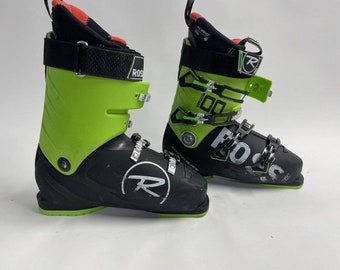The image depicts a pair of black and green rollerblades positioned against a light gray background. Each rollerblade features a top strap and another green strap on the front. The rollerblade on the left has a white letter "R" encircled, while the one on the right bears the brand name "ROSS" in white letters. Both rollerblades also include metal parts integrated into the straps and multiple hook-like structures around them. Additionally, the lining at the top of the rollerblades appears to include shades of orange or red. The background remains solid gray, with light creating slight variations in the hue.